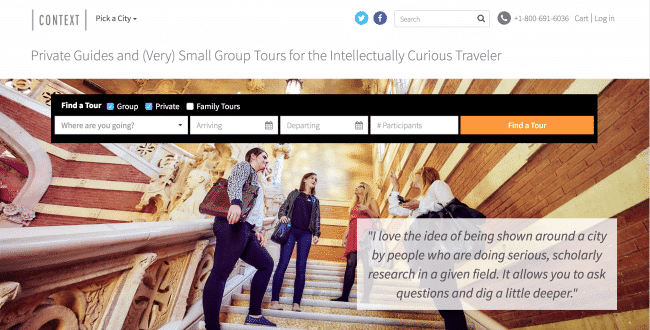The image displays a webpage featuring an assortment of options for booking a tour. At the top, there is a header that reads "Context" with a prompt "Pick a city" accompanied by a drop-down menu. Below this, there's a search bar and a call icon with the phone number "1-800-691-6036," followed by "Cart" and "Login" options. 

The main title on the page states, "Private guides and very small group tours for the intellectually curious traveler." Below, there are options to find a tour categorized into "Group," "Private," or "Family" tours. The "Group" and "Private" options are highlighted, whereas the "Family" tours option is not checked and appears in white. 

Further down, there is text prompting the user with "Where are you going?" accompanied by drop-down menus for "Arriving," "Departing," and "Number of participants." The "Find a tour" button is prominent.

The lower part of the image features a photograph of four women standing on the steps of what looks like a museum. They are casually dressed in jeans and t-shirts, each carrying a purse. The women are split into pairs, each group of two standing on either side of the staircase, engaged in conversation and gesturing animatedly. A caption below the photo reads, "I love the idea of being shown around a city by people who are doing seriously scholarly research in a given field. It allows you to ask questions and dig a little deeper." 

Overall, the setup of the webpage and the imagery emphasize a scholarly and engaged touring experience, tailored for small groups and individuals seeking deeper insights.